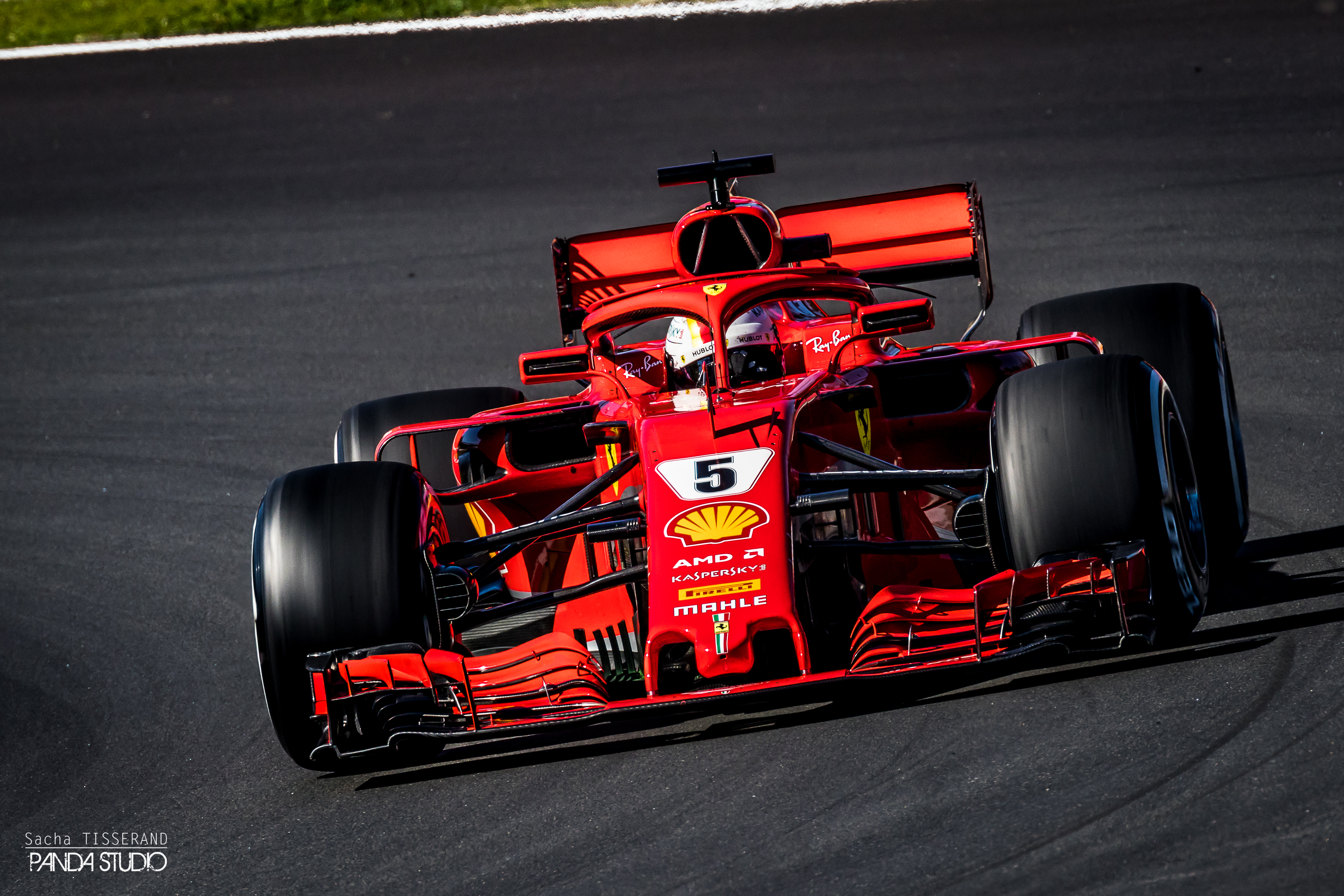The image showcases a striking red Formula Racing car, distinguished by its number 5 emblazoned in black. The car features massive black tires and multiple sponsor logos, including Shell with its yellow emblem on a red background, AMD, and MAHLE. A small Ferrari logo, the iconic prancing horse, is also visible towards the bottom. The car, equipped with a rear wing, is set on a dark gray racetrack, with a hint of curvature in the background. The driver is visible, wearing a white helmet adorned with various designs. In the bottom left corner of the image, the text "Sasha Tisserand" is separated by a line from “Panda Studio.” A narrow strip of grass can be seen running from the top left to the middle top section of the image.